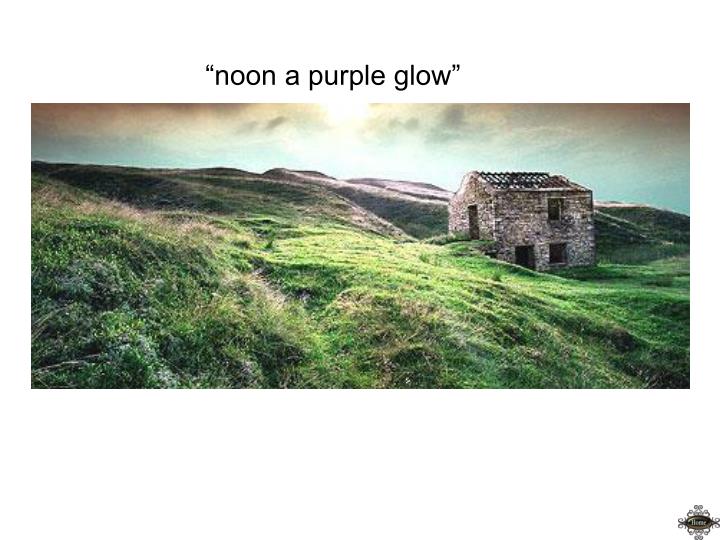The image, set against a clean white background, features intriguing black text at the top reading "noon, a purple glow" and white text at the bottom that spells "home" on a black backdrop bordered by squiggly black lines. Central to the image is an unfinished brick house, devoid of windows or doors, though another account mentions a doorway and three windows on the right side, illustrating some discrepancies in the observation. The rooftop is partially constructed with some missing tiles. This structure is situated on vibrant rolling hills, which display a palette of black, gray, white, yellow, and green hues, with particularly lush, green grass around the home. The sky overhead is a mix of blue and orange tones, filled with white clouds and illuminated by the sun's rays breaking through, suggesting a bright noon setting. The scene resembles a quaint, European countryside, possibly likened to an Irish landscape, and could be interpreted as a painting or a drawing.